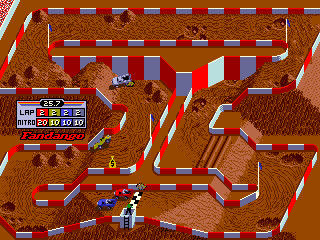This image, potentially taken from an old video game such as Minecraft or another classic racing game, showcases a vibrant racing scene. The racetrack is distinctly lined with alternating red and white squares, creating a striking visual boundary. Two cars are battling it out on the track, with one car painted a vivid red and the other a light blue. At the top of the image, a title "Fandango" is prominently displayed, along with crucial race information indicating that all cars are currently on lap 2, accompanied by their respective scores. The graphics exhibit a blend of 2D and 3D elements, characterized by a rudimentary, pixelated style typical of early video games. The minute details are challenging to decipher due to the primitive graphical quality, reinforcing its vintage aesthetic.